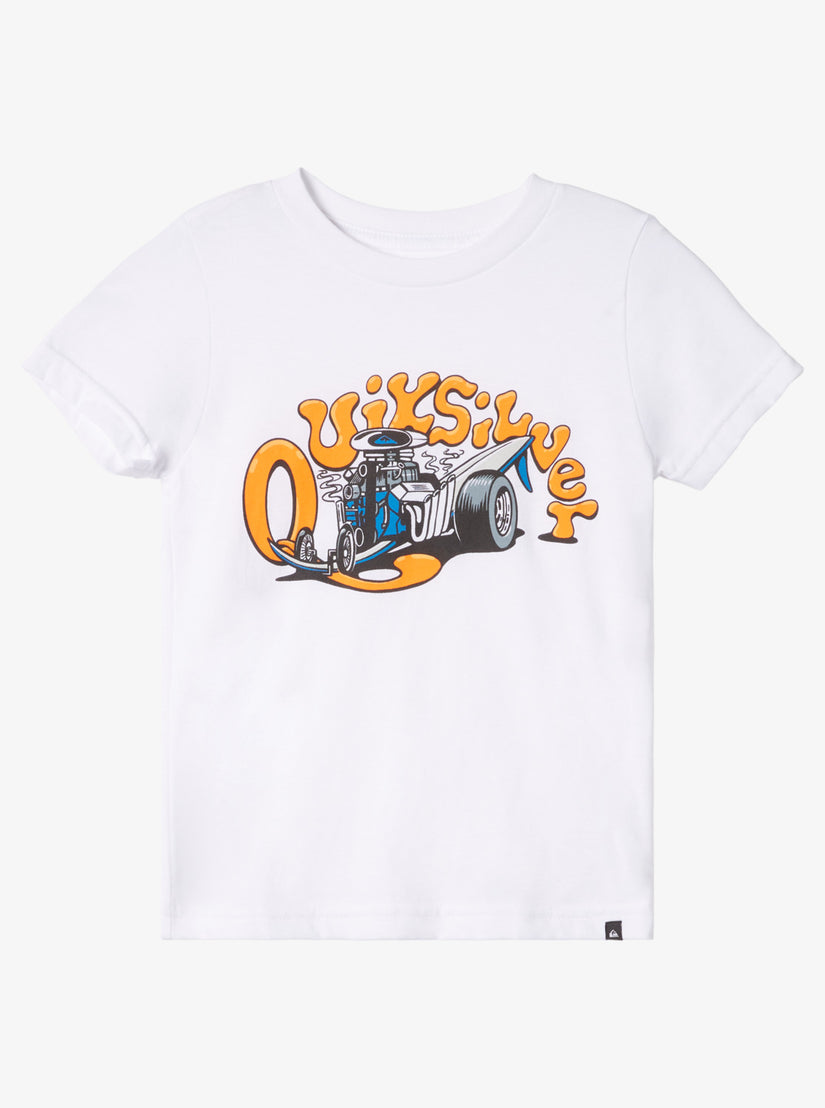This image features a vertically aligned, rectangular shot, showcasing a white t-shirt laying in the center against a white background, which is slightly duller than the vibrant, pristine white of the t-shirt itself. The short-sleeve, crew neck t-shirt is precisely laid out and well-lit, emphasizing its clean design. 

Dominating the front of the t-shirt is a graphic that reads "quiksilver" in stylized, curvy orange bubble letters that arch upwards and then downwards. The letters are a mix of uppercase and lowercase, with the "Q" being notably larger. Below this text is a cartoony depiction of a unique, surfboard-inspired vehicle. The vehicle has a large rear wheel, a stem that curves upward into two tiny front wheels, and a surfboard-like body complete with a downward-pointing fin and a central engine block adorned with the Quiksilver logo. The color scheme of the vehicle consists of black, white, and a bright medium blue, with intricate detailing of pipes and machinery around the engine.

In the lower right-hand corner of the t-shirt, there is a small black tag sewn in, featuring a white Quiksilver logo. This tag adds a subtle yet recognizable branding element to the already distinctive design.